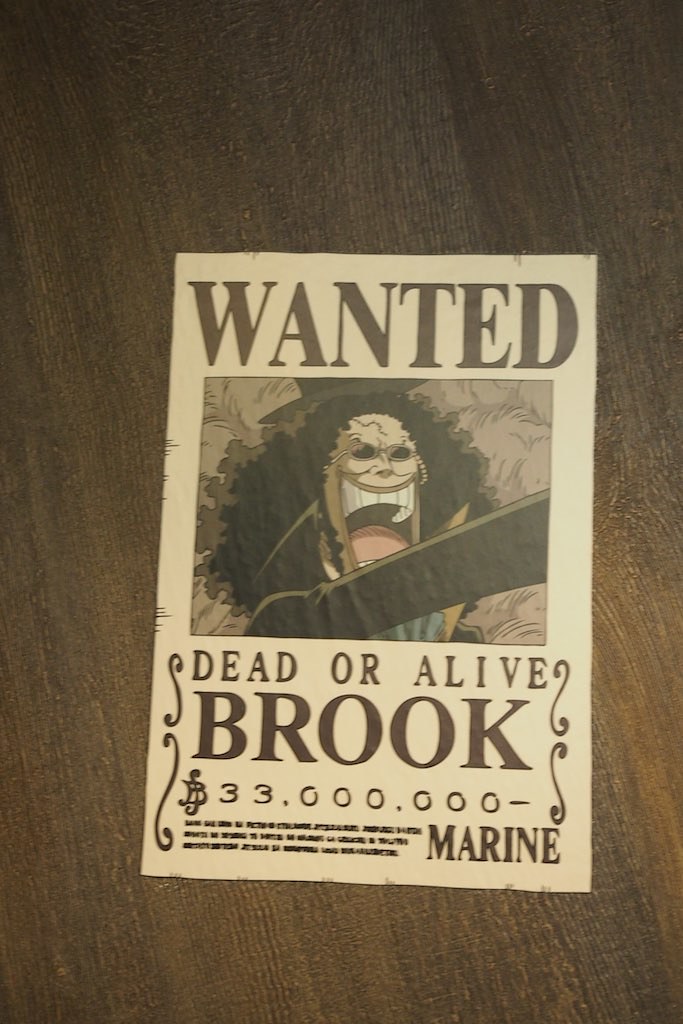The image depicts a detailed, cartoon-style WANTED poster that features intricate design elements. The poster is printed on an off-white piece of paper, which is placed on a dark wooden surface. The poster is dominated by the word "WANTED" in bold, capital letters at the top. Beneath it is a cartoon drawing of a character that resembles a rock-and-roll star; he has long, frizzy black hair, thin dark glasses, and is wearing a hat. The character's mouth is open wide, revealing large teeth, and his skin has a tan tone with red or pink inside the mouth. Below the illustration, in dark brown lettering, it states "DEAD OR ALIVE BROOK" followed by "33,000,000" indicating a thirty-three million dollar bounty. The word "MARINE" is inscribed at the bottom right corner. The poster features some decorative squiggly line designs flanking the main text, further emphasizing its cartoonish, somewhat menacing appearance.